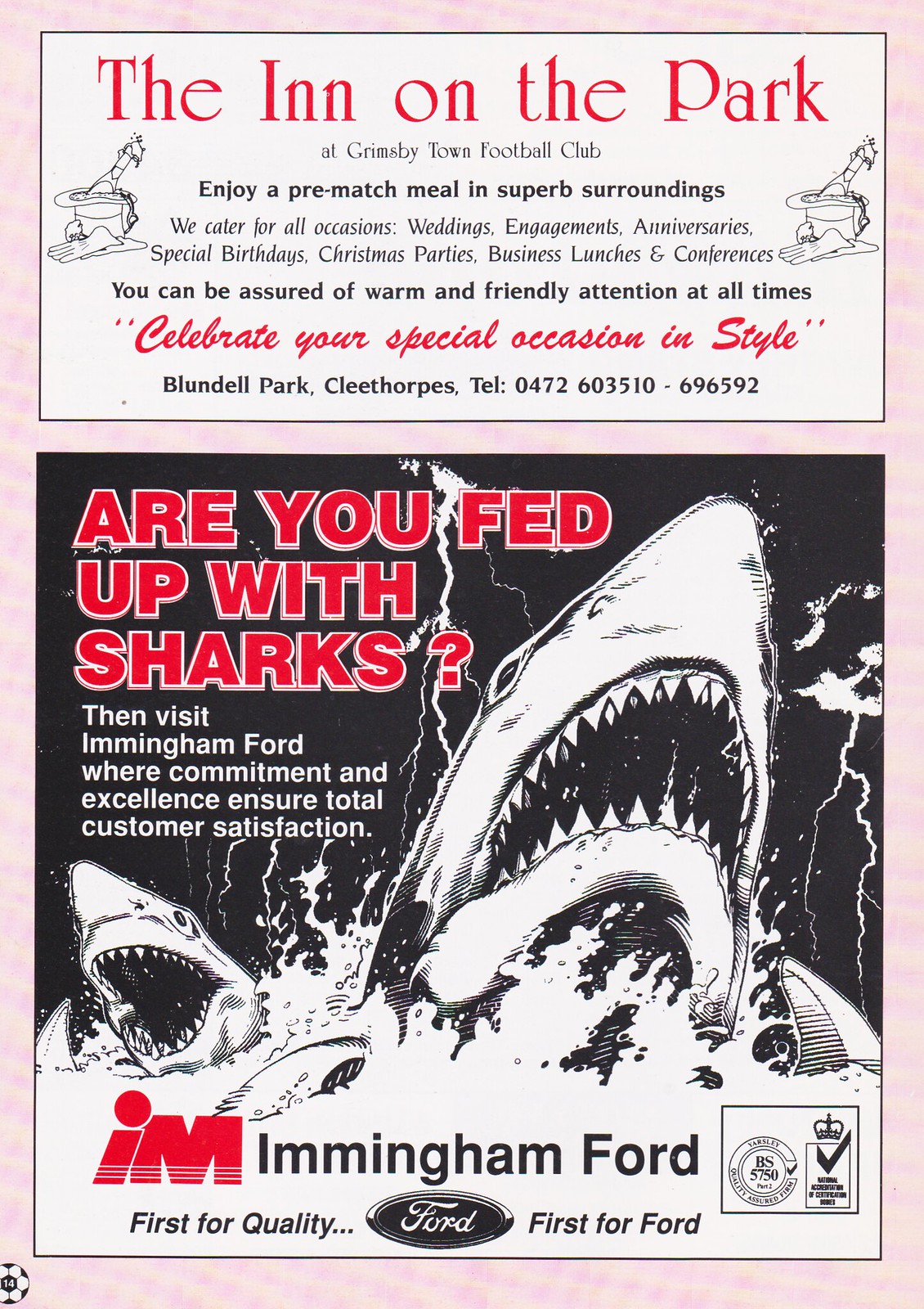This is an advertisement page reminiscent of a magazine spread with a pink background, featuring two distinct adverts. At the top, in bold red lettering against a white backdrop, it promotes "The Inn on the Park at Grimsby Town Football Club." The advertisement invites patrons to enjoy a pre-match meal in superb surroundings and caters to various occasions such as weddings, engagements, anniversaries, special birthdays, Christmas parties, business lunches, and conferences. It assures warm and friendly attention at all times, with the slogan "Celebrate your special occasion in style" in red letters, followed by the address and phone number in black. The ad is complemented by charming drawings, including gloves and champagne in a bucket, enhancing the celebratory ambiance.

Below this, there is a contrasting, eye-catching advertisement in predominantly black and white with red highlights. It asks, "Are you fed up with sharks?" in vivid red text, promoting the Immingham Ford dealership. The ad, featuring hand-drawn images of menacing sharks with wide-open mouths and sharp fins, emphasizes the dealership's commitment to excellence and total customer satisfaction. It concludes with the slogans "Immingham Ford – First for Quality" and "Ford – First for Ford," alongside a quality assurance seal with a crown, underscoring the dealership's dedication to high standards.